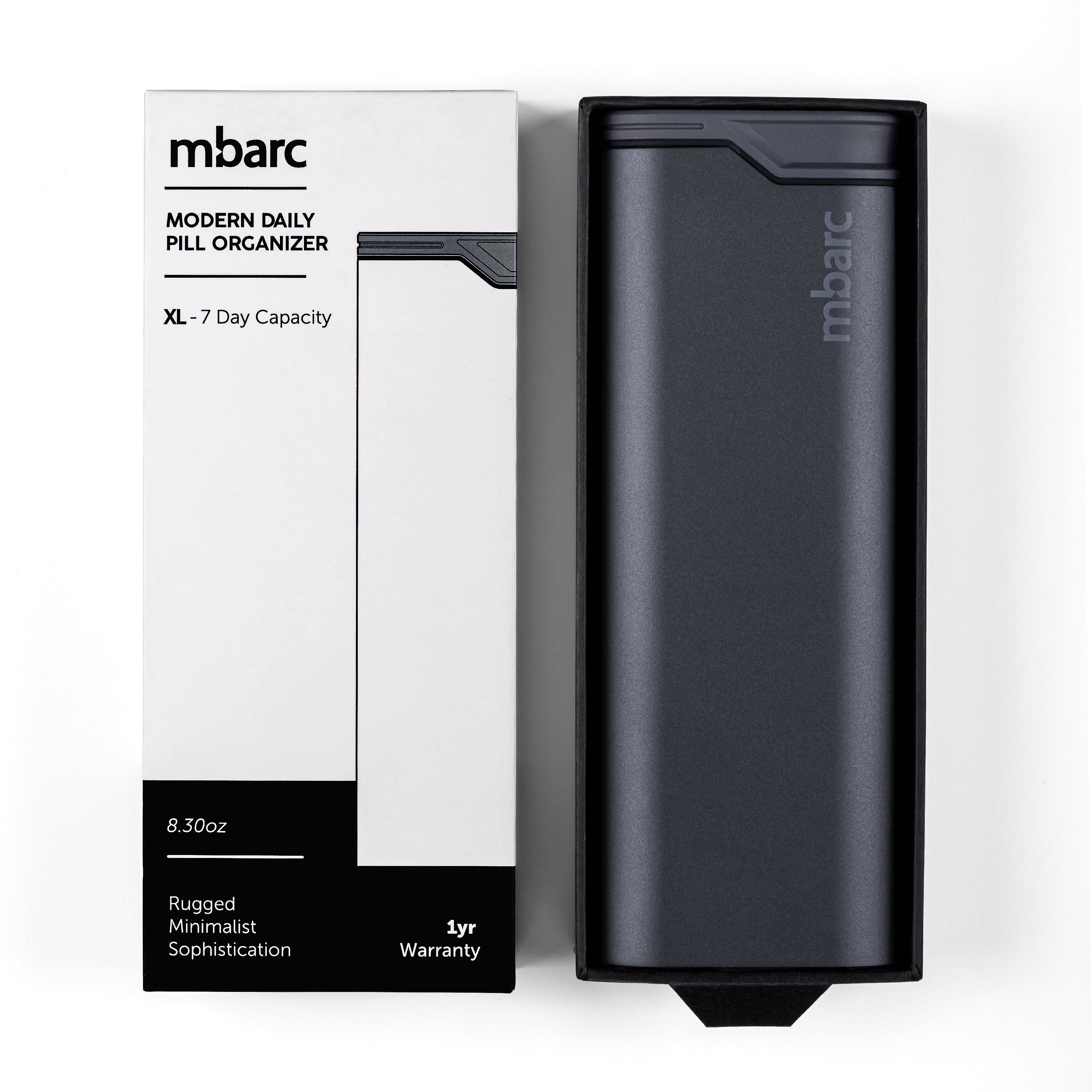The image displays a sleek and modern daily pill organizer branded as Embark. The product is showcased alongside its packaging, which is a rectangular box predominantly white with a black lower section. The top of the box features the brand name "Embark" in a bold sans serif font, followed by the description "Modern Daily Pill Organizer." It then identifies the product as "XL, 7-day capacity, 8.30 ounces," and highlights features such as "rugged minimalist sophistication" and a "one year warranty." The pill organizer itself, placed next to the box, is a dark gray or black rectangular object with rounded edges. It is made from a rugged material with a matte finish and has the brand name "Embark" embossed or printed towards its top. The organizer has a smooth surface and a design that suggests a balance between durability and modern aesthetic.